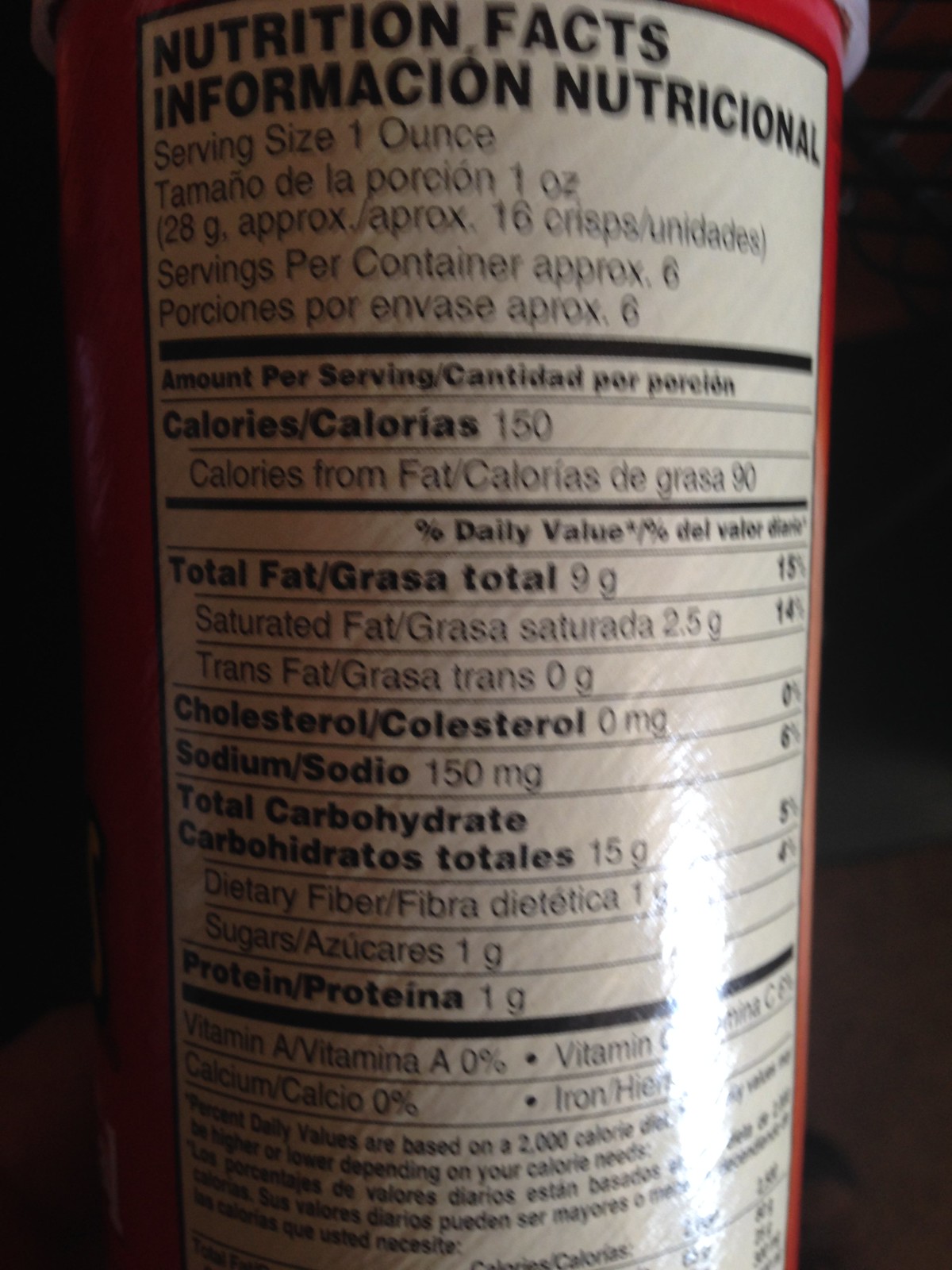The image showcases a cylindrical bottle prominently positioned in the center against a blurry, dark background. The label on the bottle features text in black on a white backdrop. At the top of the label, the words "Nutrition Facts" are clearly discernible. Just below this, the label displays the Spanish phrase "Información Nutricional." Further down, the label specifies the serving size as "1 oz." The overall image quality is notably poor, characterized by blurriness and fuzziness. However, the essential details on the label remain legible despite the low resolution.